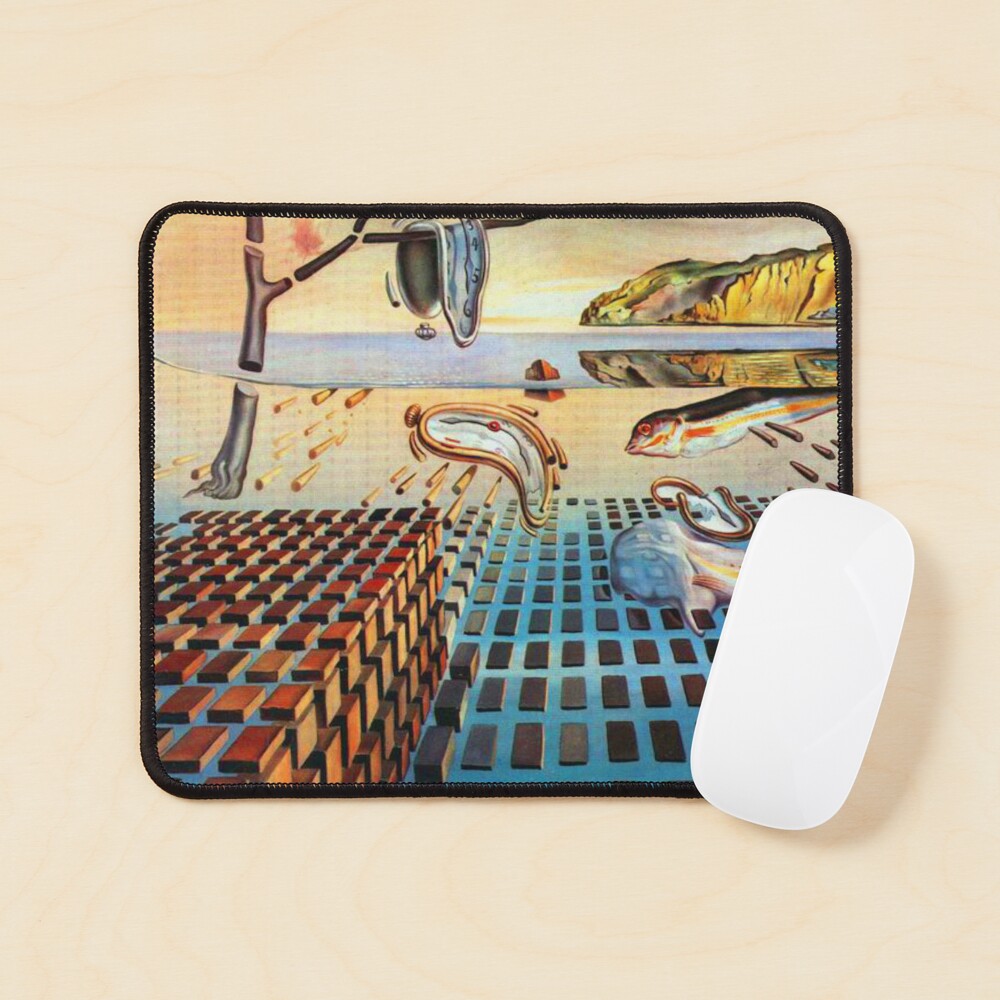A top-down photograph captures a mouse pad featuring Salvador Dali's surrealist painting, "The Disintegration of the Persistence of Memory." The mouse pad is bordered in black and rests on a tan, wood-finished surface, where the faint grain of the wood is visible. On the bottom right corner of the mouse pad, there is a white computer mouse.

The Dali painting on the mouse pad portrays an avant-garde scene with melting clocks, fragmented blocks, and other surreal elements. At the center, a melting clock is prominently displayed. Beneath the clock, rows of brown blocks float in water. A segmented tree with another melting clock draped over one of its branches is positioned at the top left corner. A gray fish with a yellow and orange stripe swims in the water on the right side. The right side of the artwork also features a rocky formation, part of which appears mountainous with hues of brown, green, and purple, reflected in the water's surface. The composition, rife with abstract and surreal details, captures the essence of Dali's dreamlike imagery.